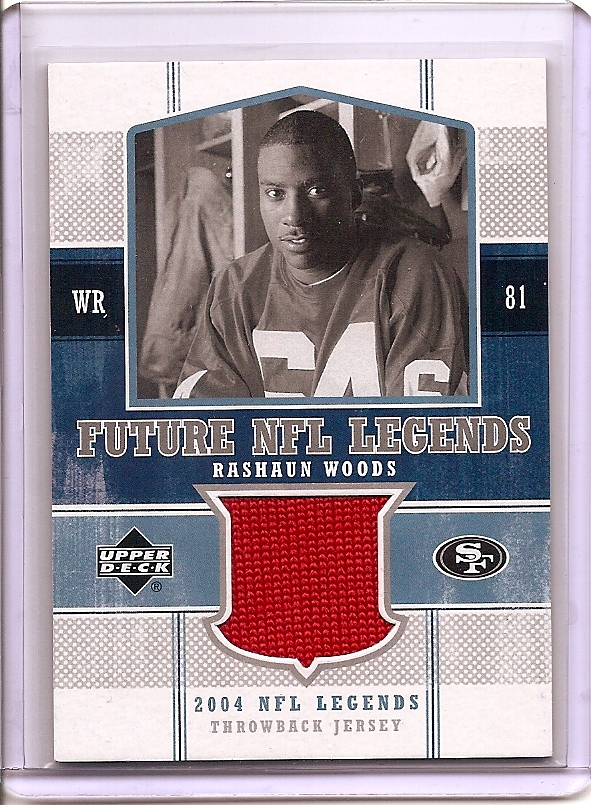This image features a football trading card encased in a clear protective sleeve. The card displays a black and white photograph of Rashawn Woods, a young man with a short haircut wearing a jersey with the number 81. The top of the card has "WR" in white letters to the left of the photo and "81" to the right. Below the image, in gray font, it reads "Future NFL Legends," followed by Rashawn Woods' name in white font. In the middle of the card is a blue line with a red badge, displaying "Upper Deck" on the left and the "SF" San Francisco 49ers logo on the right. Additionally, there appears to be a small viewport containing a piece of fabric, possibly from Woods' jersey. At the very bottom, in small blue text against a white background, the card says "2004 NFL Legends Throwback Jersey."